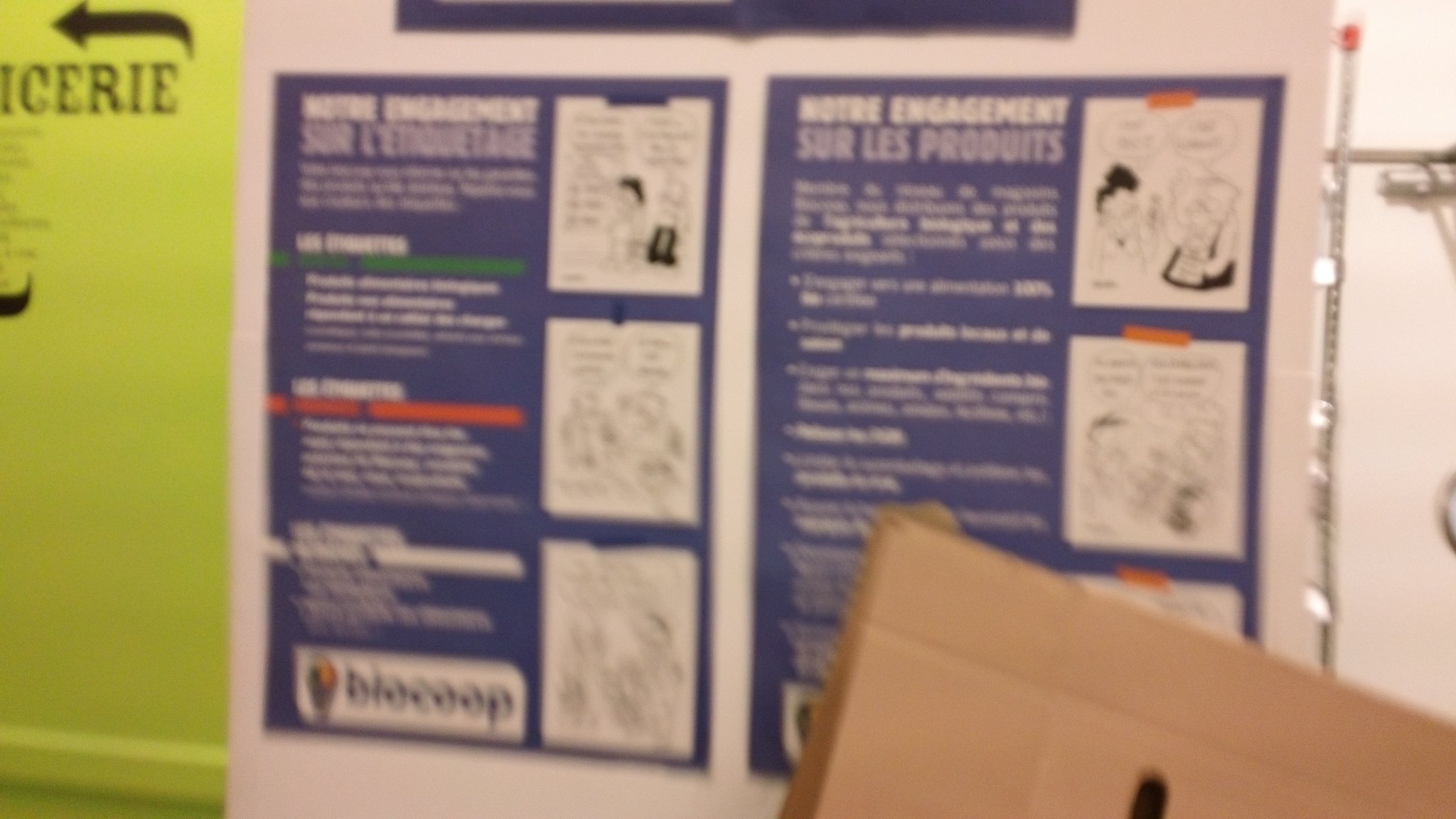A series of posters adorn a white wall, creating a visually engaging display. On the far left, a yellow poster features bold black text at the top, standing out against its bright background. Adjacent to the yellow poster, and also to the right, are blue posters, one on each side. In the forefront, a cardboard-brown poster captures attention with its unique texture. Though slightly out of focus, the bottom left corner of this poster appears to contain the word "Biocoop." The central theme of the brown poster includes three detailed illustrations and a prominent tower situated on the right-hand side. The text on these posters is in a different language, adding an element of cultural intrigue to the arrangement.